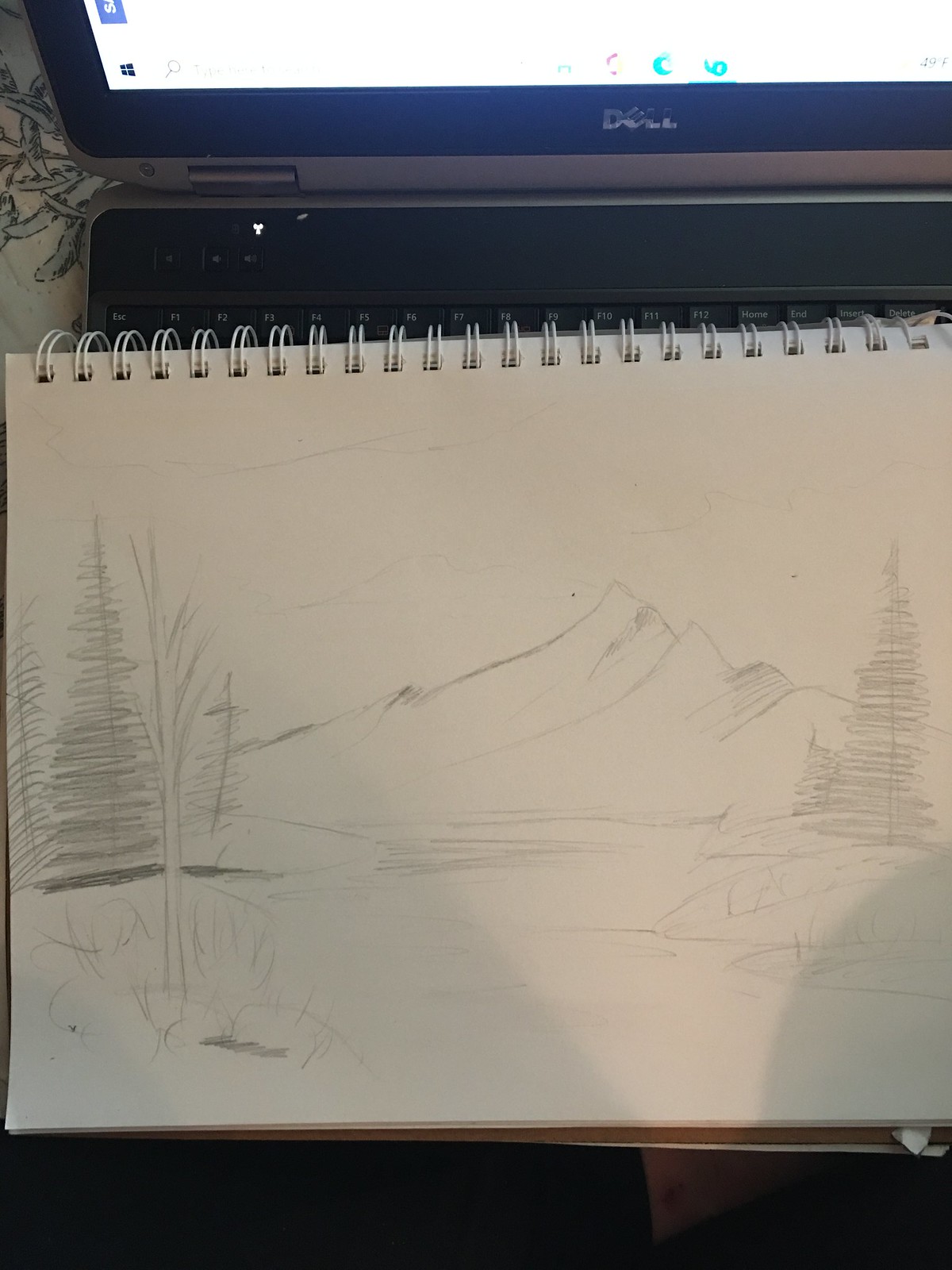The photograph features a wire-bound sketchbook resting on the keyboard of an open laptop. The visible portion of the laptop includes the upper part of the keyboard and the bottom 10% of the screen. The sketchbook itself has white paper and white binding. The page currently displayed showcases an intricately detailed pencil drawing of a serene winter landscape. Central to the composition is a mountain positioned slightly to the right, its snowy peak contrasting against the darker pencil strokes. Flanking the mountain are evergreen trees, with one on each side of the drawing. Adjacent to the pine tree on the left is a barren tree stripped of its leaves, adding a stark element to the wintery tableau. In the foreground, a body of water is depicted, with rocks scattered along the right edge, lending a sense of depth and realism to the scene. A shadow, presumably cast by the photographer, partially obscures the detailed sketch, adding a touch of mystery and human presence to the image.